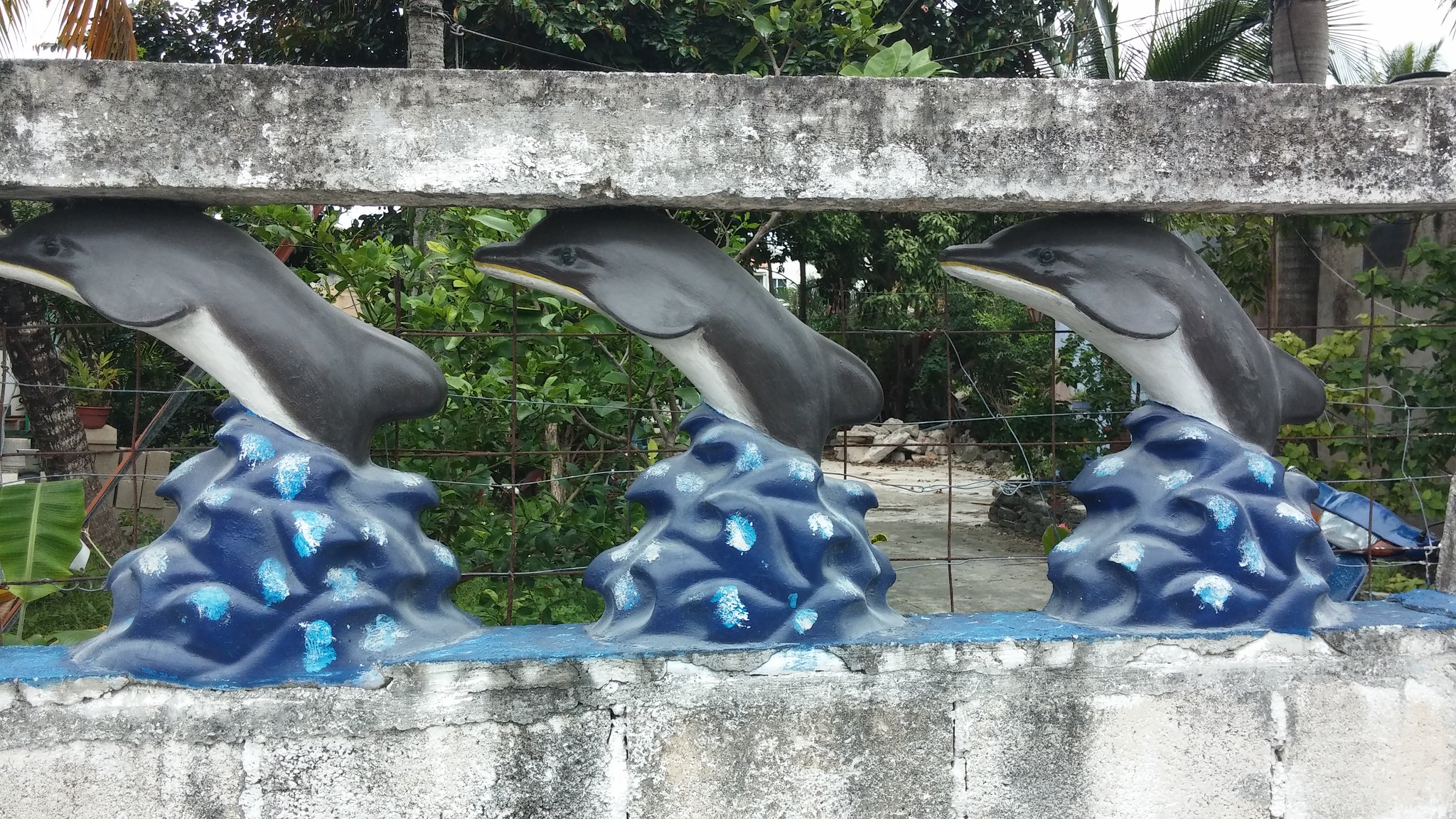In the photograph, a detail shot captures an ornamental fence made of aged concrete marked by black and white splotches. Central to the image are three sculpted dolphins, each positioned in profile view and facing left. These dolphins, with black backs and white underbellies, appear to be leaping out of an artistically sculpted blue wave featuring detailed contours and white splotches to mimic frothy water. The dolphins sit between two weathered, horizontal stone planks, which boast numerous cracks and breaks. Behind the dolphins, there is a rusty orange metal wire fence, with verdant green trees and bushes, possibly part of a park, visible in the background. The stone path or possibly water lies beyond, all beneath a slightly overcast but bright sky, indicating that the photograph was taken on a sunlit day.